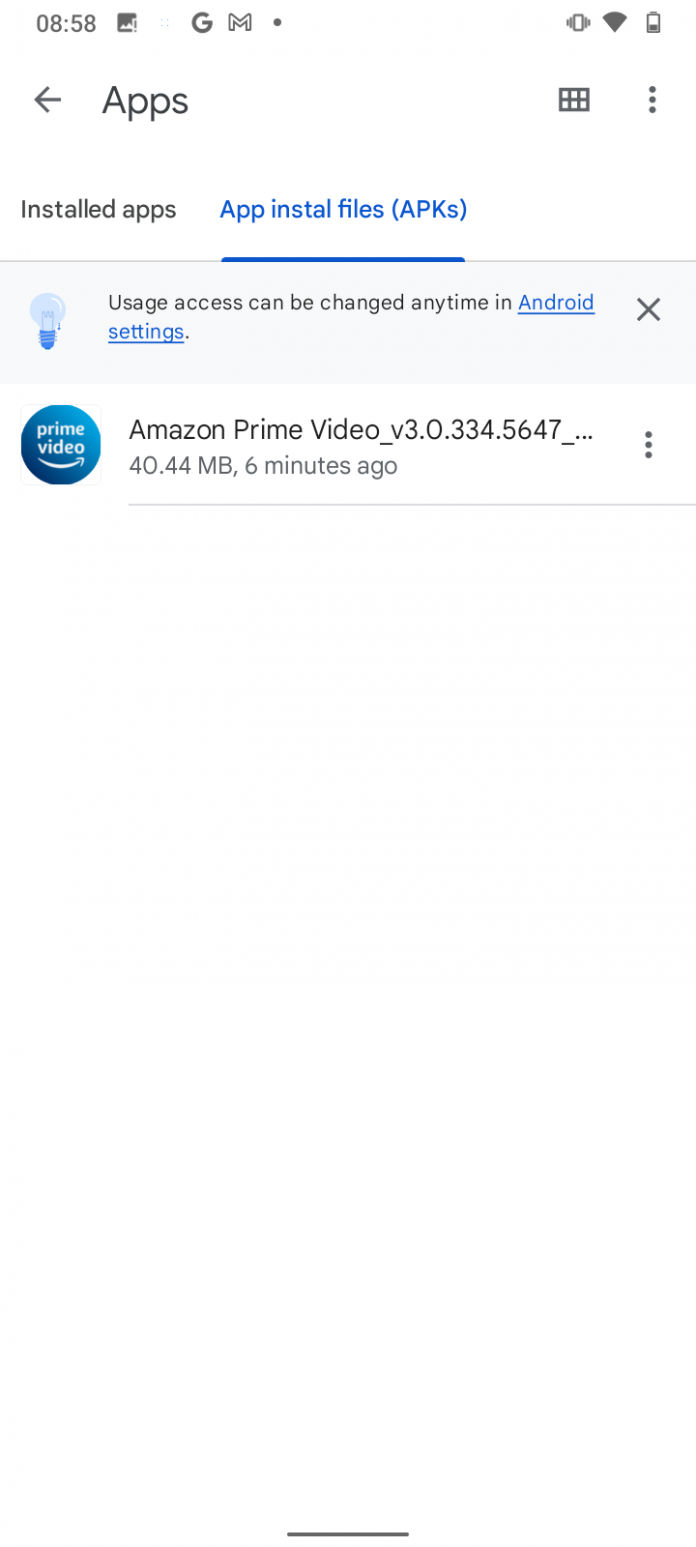This cropped screenshot displays the "Apps" tab on a smartphone with a white background. In the top left corner, the word "Apps" is written in black letters with a left-pointing arrow next to it. Directly below, there are two tabs labeled "Installed Apps" and "App Install Files (APKs)," with a blue underline indicating that the "App Install Files (APKs)" tab is currently selected. 

Underneath, two notification boxes are present. The first box contains a message: "Usage access can be changed anytime in Android settings," with "Android settings" hyperlinked in blue. To the right of this box, there is an "X" icon for closing the notification, and to the left, a blue light bulb icon.

The next section shows the Amazon Prime Video app information. On the left, there is the Amazon Prime Video logo. In the center, the text reads "Amazon Prime Video" followed by the version number. Below this, it displays the file size and a note indicating the app was updated 6 minutes ago. To the right, there is a vertical three-dot icon for accessing more options.

At the very top of the screenshot, the phone's status bar is visible. It displays the current time on the left, along with the Google icon and another system icon. On the right side, the icons indicate that the phone is on silent mode, connected to Wi-Fi, and shows the current battery percentage.